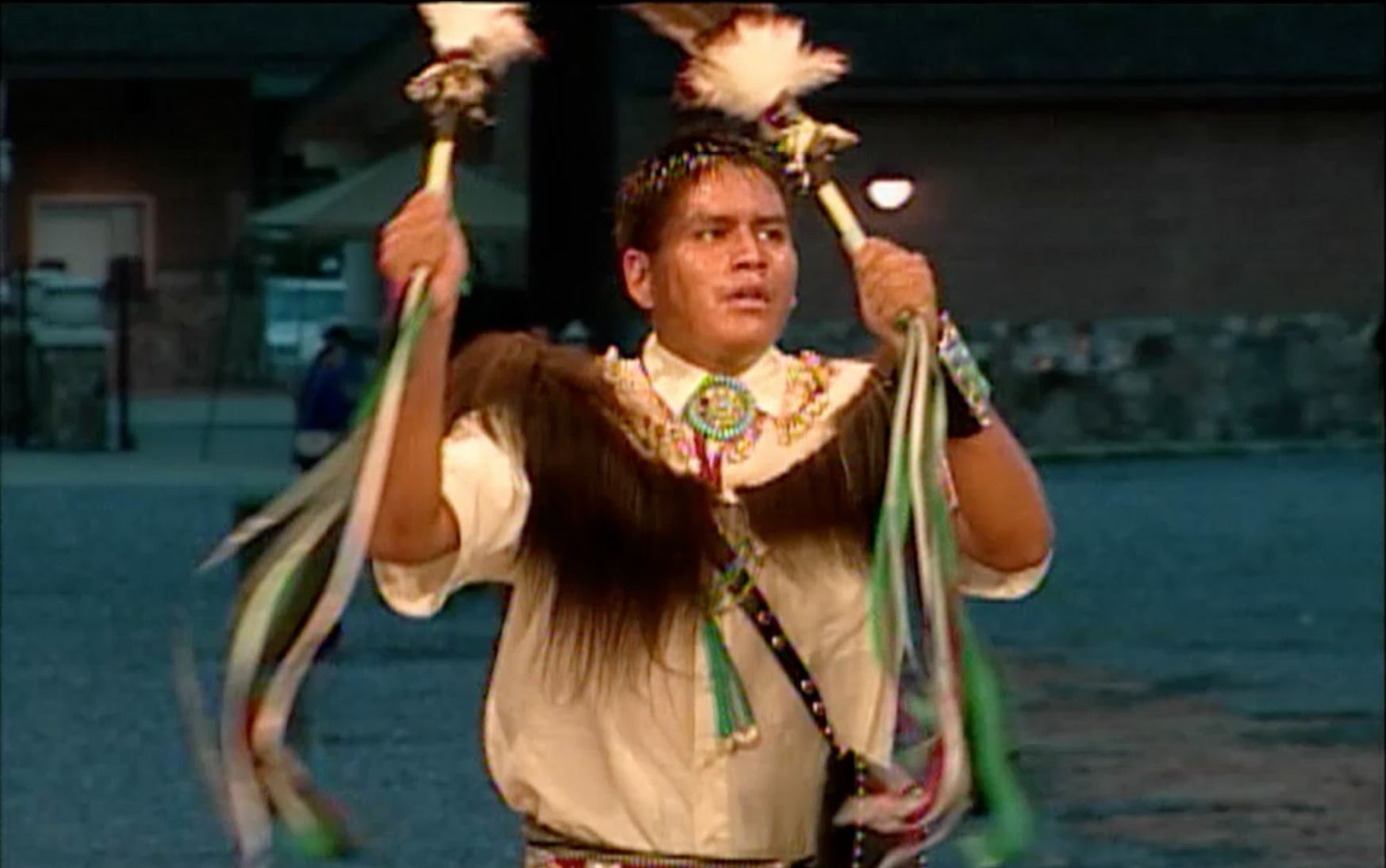The photograph captures a young man, possibly of Latin or Native American descent, engaging in a traditional dance at night. He is dressed in a modern button-up short-sleeve shirt that forms a contrasting backdrop to the various traditional elements of his attire. Draped across his chest is a piece of animal fur, and he wears a circular decorative necklace resembling a dreamcatcher, as well as a bolo tie. His wrists are adorned with bracelets, and he has a choker around his neck. In each hand, he holds a baton-like rattle, adorned with feathers and colorful streamers in green, white, and red, which appear to blur from rapid movement. A metal-studded satchel or sack is slung over his shoulder, adding to the eclectic mix of his outfit. His hair is possibly accessorized with feathers, hinting at cultural significance. The background features the indistinct outline of a suburban house and other outdoor elements, making the focal point his dynamic presence and attire, as he performs this energetic and captivating dance.